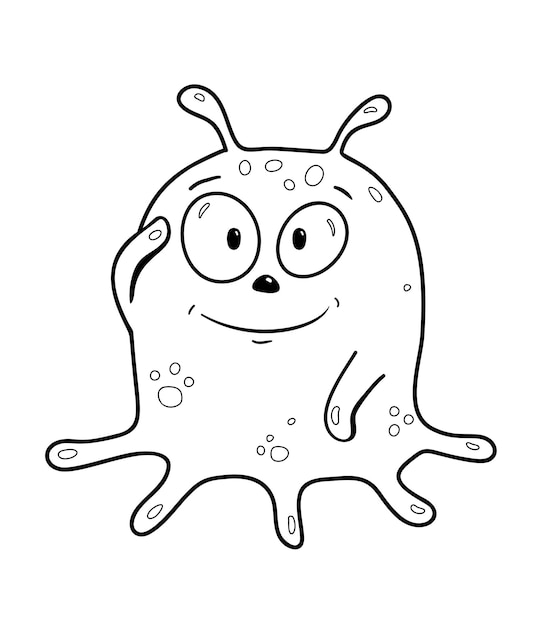This image is a pen and ink cartoon of an anthropomorphic, blob-like creature that combines features reminiscent of a Japanese pumpkin squid and a cute amoeba. The creature has a bulbous top with two antenna-like projections adorned with circular patterns. It sports two large oval eyes, the left being larger, each set below expressive little eyebrows. The creature's nose is tiny and pebble-shaped, and it has a cheerful smile accentuated by two small dimples.

It has seven visible arm-like appendages; one arm is raised near its eye, as if saluting, while another rests by its side. The remaining five limbs extend to the ground, appearing to support the creature's weight. These appendages are covered with round spots, which also scatter across its amorphous body, lending it a playful and endearing appearance. With its simple, line-drawn style, this creature evokes the charm of a coloring book image, poised somewhere between a puppy dog and an octopus.